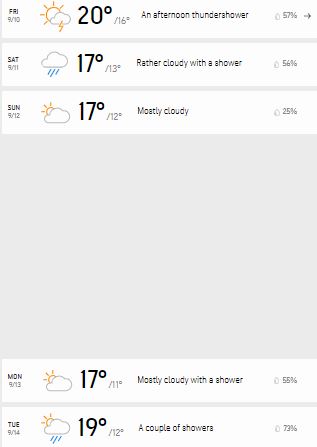A detailed weather forecast is displayed on a smartphone screen, presenting a clear layout of the upcoming days. On the left side, the day and date are prominently shown, such as "Friday 9/10", "Saturday 9/11", and "Sunday 9/12". Accompanying each date is a weather icon that visually represents the forecast, such as an afternoon thundershower icon, a cloud with blue streaks for rain, and a sun partially hidden by clouds.

For Friday, September 10th, the forecast predicts an afternoon thundershower, with temperatures reaching a high of 20 degrees Celsius and dropping to a low of 16 degrees Celsius. There is a 57% chance of rain. On Saturday, September 11th, the weather is expected to be rainy, depicted with a cloud and blue streaks. The high is forecasted at 17 degrees Celsius and the low at 13 degrees Celsius, with a 56% chance of rain. Sunday, September 12th, shows the sun obscured by clouds, predicting mostly cloudy conditions, a high of 17 degrees Celsius, a low of 12 degrees Celsius, and a 25% chance of rain.

The middle area of the screen is filled with a gray, empty square, possibly indicating a loading or unavailable section. Below this gray area are two more sections that continue the weather forecast, although specific details are not provided in the description. The detailed presentation ensures all relevant weather information, including temperatures, conditions, and precipitation chances, are easily accessible and visually organized.